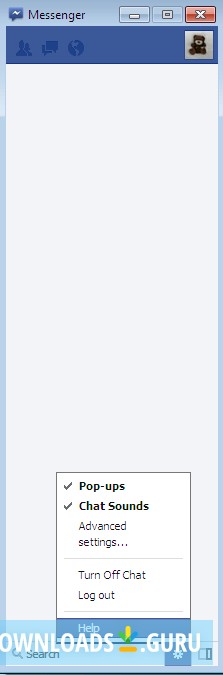The image depicts a vintage, pop-out window of the classic Facebook Messenger app. The window is framed with an ice-blue color along the top, left, right, and bottom edges. At the top left corner, there's a chat icon featuring a lightning bolt inside. Right next to this icon, the word "Messenger" is displayed in black font. Adjacent to the text, on the top right, are three familiar window control buttons: minimize, maximize, and a red-and-white "X" for closing the window.

Below the header, on the left side, are tabs for friends, messages, and a web icon. Positioned opposite these tabs, a small, brown teddy bear image can be seen. Dominating the center of the window is a blank screen, suggesting that no active chats are currently displayed. At the bottom of this screen is a search bar for user convenience.

Additionally, a pop-up is visible with several options: "Pop-ups allowed," "Chat sounds allowed," "Advanced settings," "Turn off chat," and "Log out," providing quick access to various functionalities and settings of the messenger app.